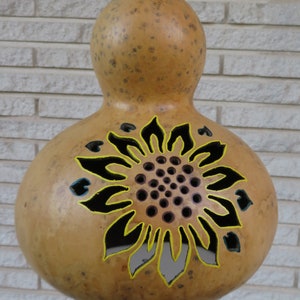This photograph features a unique ceramic piece set against a backdrop of a white brick wall. The ceramic structure resembles a whimsical snowman or a smushed bowling pin, with a rotund, round base and a much smaller, spherical top. The ceramic surface is predominantly a light brown color with occasional dark brown splotches, giving it a somewhat natural, rustic appearance. 

A decorative flower is prominently featured on the lower, largest part of the piece. This flower has a center of faint pink, filled with black dots arranged in concentric circles. The petals surrounding the center are black, each meticulously outlined in a thin yellow line. Additionally, there are small punch-outs creating decorative leaf patterns at the top of the large spherical base, enhanced with subtle blue lines around them. This intricate detailing lends the piece a charming and handcrafted aesthetic.